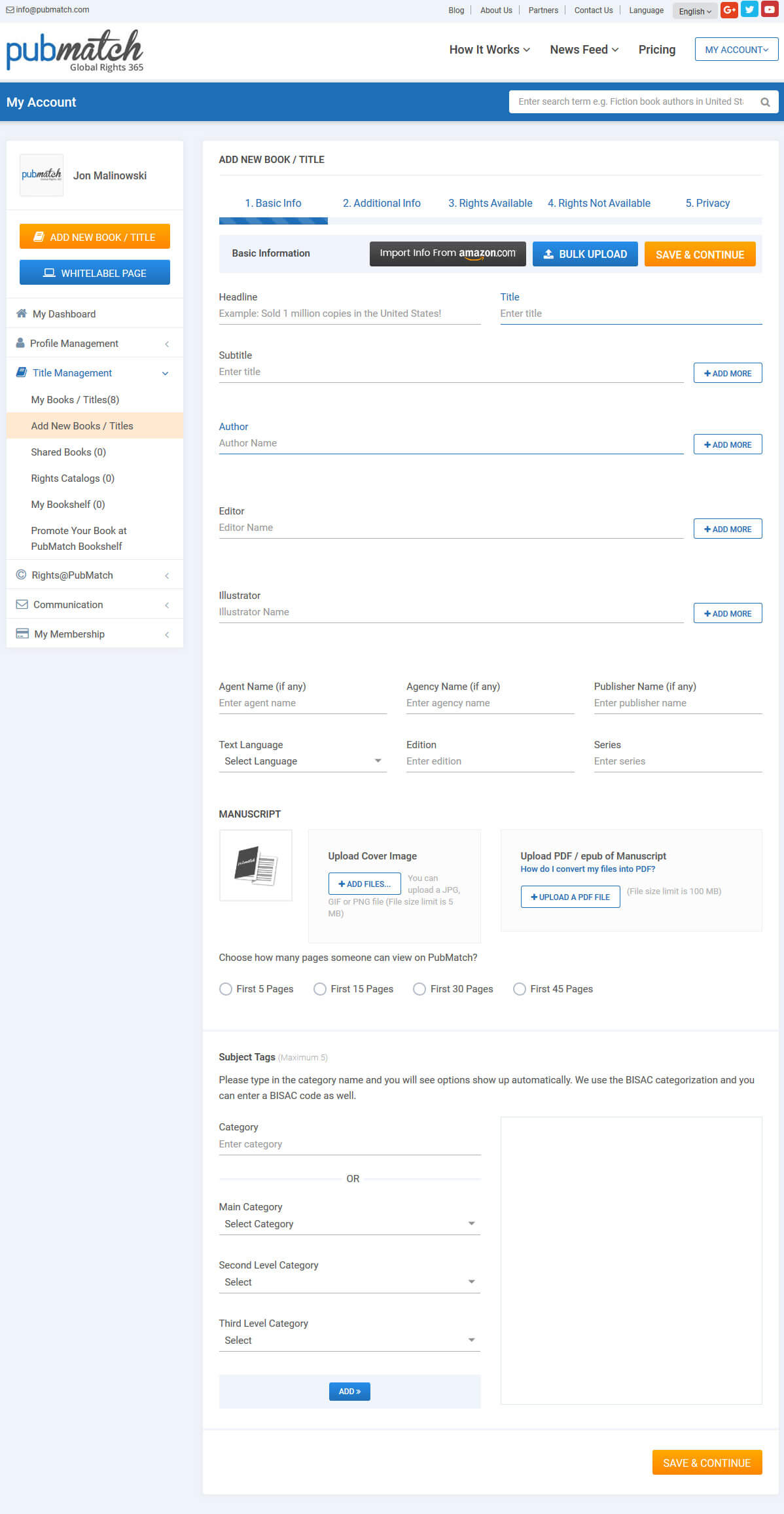The image features a user interface from a PubMatch.com page. The layout includes a light gray border encompassing the left side of the page. At the top left corner is a black envelope icon with the email "info@pubmatch.com" in black text. Spanning across the top are several navigation tabs in black text: "Blog," "About Us," "Partners," "Contact Us," and "Language." 

Adjacent to these tabs, set on a gray background, is the word "English" in black, accompanied by icons for Google Plus, Twitter, and YouTube. Below the header, the background transitions to white, showcasing the site’s logo: "Pub" in blue and "Match" in black. The tagline "Global Rights 365" appears in black text beneath the logo.

Further below, the navigation menu continues with black text: "How it Works," "News Feed," and "Pricing." At the far right, "My Account" is highlighted in blue. 

The left-hand side features a blue sidebar with "My Account" written in white at the top. Below this, there is a white search box with placeholder text in light gray: "Enter search term e.g., fiction book authors in the United St…" followed by a gray magnifying glass icon. In the blue sidebar, "John Malinowski" appears in black text at the top of a rectangular section.

There are two additional rectangles beneath this: an orange and white one labeled "Add New Book/Title" and a blue and white one labeled "White Label Page." The dashboard menu follows, with items listed in black text: "My Dashboard," "Profile Management," and "My Books/Titles (8)." 

Highlighted in blue is "Title Management," followed by additional options in black: "Add New Book/Title" (set against a light orange background), "Share Books," "Rights Catalog," "Bookshelf," and "Promote Your Books at PubMatch." 

Lower in the sidebar, there are more options in black text: "Rights at PubMatch," "Communication," and "Mind Membership."

At the top of the page, under the header, there are input fields labeled with "Headline Title," "Subtitle," "Author," and "Editor," each accompanied by an underlined space for entering information.